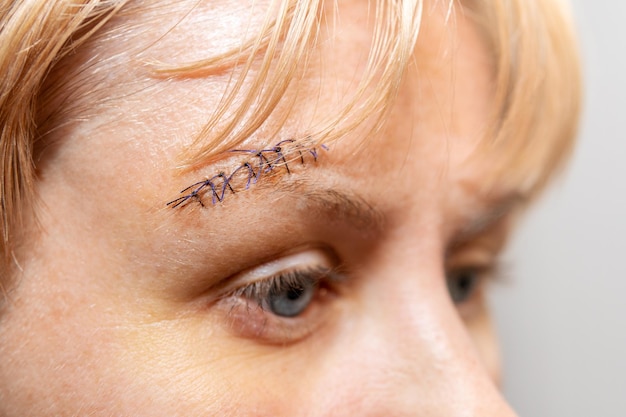This image is an extreme close-up of a young Caucasian female's forehead and upper face, captured in bright light against a solid white background. Her blonde bangs partially cover her forehead. She has striking blue or green eyes, fair skin, and blondish-brown hair. The picture distinctly shows an area above her right eyebrow with a noticeable injury that has been stitched up. The stitches are thin, black, and tightly knotted, extending across the shaved portion of her eyebrow. Reflections of the light source can be seen on her forehead, adding contrast to the detailed texture of her skin and the starkness of the injury.